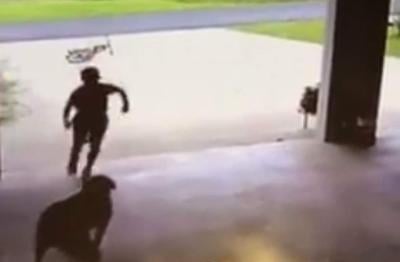A blurry image, likely from a security camera, shows a somewhat chaotic scene in a driveway. In the foreground, there's a dark silhouette of a dog facing towards a garage. A young boy, also a dark silhouette, is seen running towards the dog, seemingly in a hurry or perhaps agitated. The boy's bicycle is lying on its side a few feet back in the driveway. The right side of the image has a concrete pillar, possibly part of the house, with a hint of a bush beside it. The garage itself appears mostly empty, with only a few indistinguishable objects near the doorframe. In the background, beyond the driveway, the neighborhood street can be vaguely made out. The image captures a snapshot of what looks like a tense or hurried moment between the boy and the dog, set against the backdrop of a residential driveway.